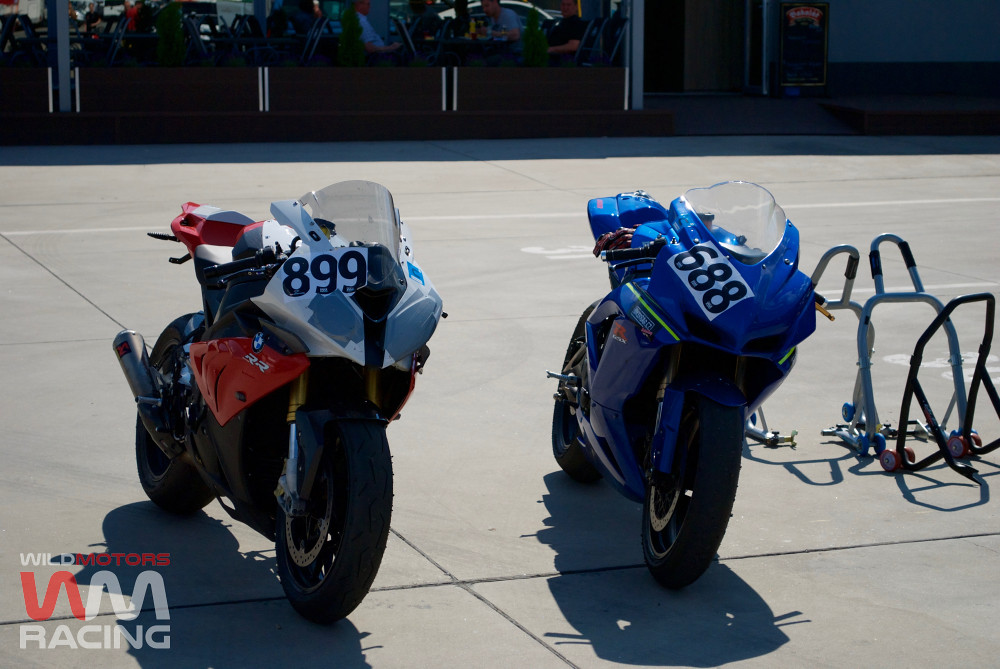This photograph captures an outdoor scene showcasing two racing motorcycles from the renowned outfit, Wild Motors Racing, as evidenced by their distinct white and red emblem with a W and M squiggle in the lower left corner. The motorcycles are positioned on a gray asphalt surface, casting shadows to the bottom left. The bike on the left stands out with its black primary color and red accents, accented by a silver front portion, and marked with the racing number 899. Interestingly, it also has some duct tape visible on its front, suggesting it may have undergone recent maintenance. The right bike, predominantly royal blue with notable lime green accents, bears the racing number 688. Both bikes, engineered for minimal air resistance, feature small windshields and lean on their kickstands. On the right side of the image, metal brackets or frames—likely used for transportation or maintenance of the bikes—can be seen. In the backdrop, the tops of buildings are faintly visible, hinting at a racetrack environment.